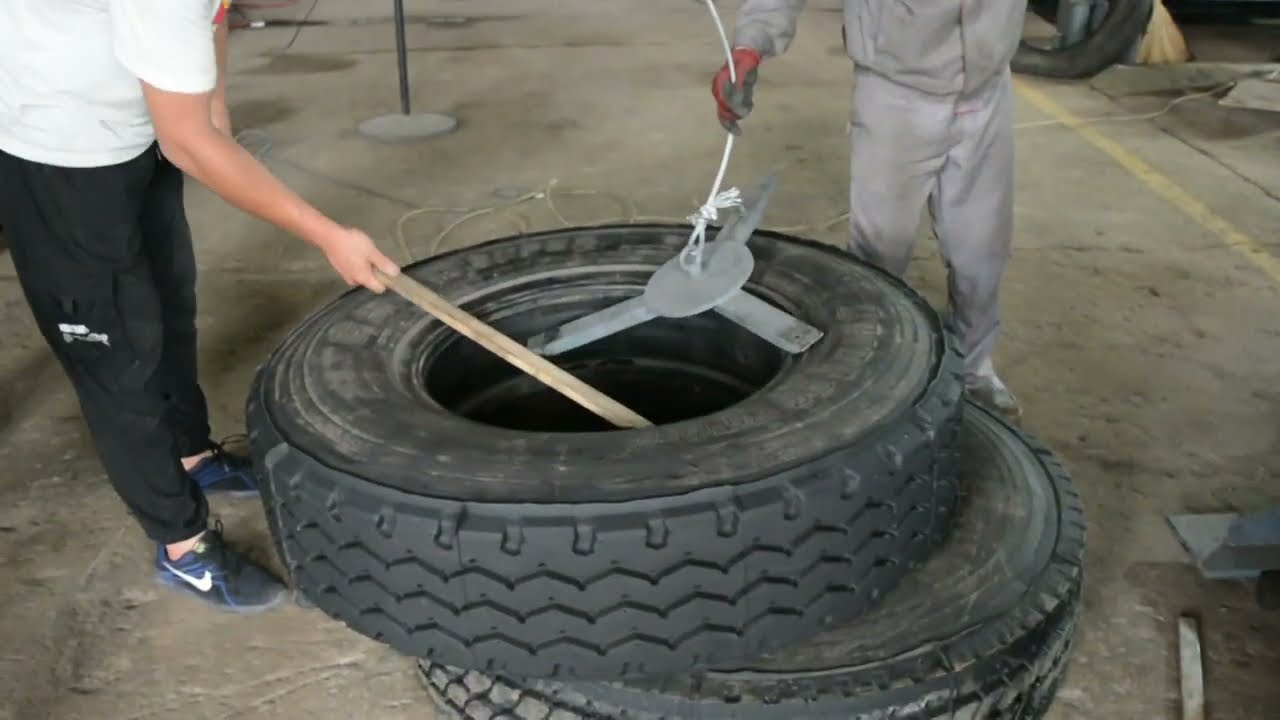The image captures a scene inside a commercial garage or body shop with a worn, dirty concrete floor. At the center of the frame are two enormous tires, one precariously stacked atop the other, slightly off-center. To the left of the tires stands a Caucasian man dressed in a white t-shirt, black pants, and blue Nike shoes. He is bent over, holding a long wooden stick that he is inserting into the center of the top tire. On the right side and a bit behind the tires is another man, dressed in a light gray tracksuit and possibly wearing a red glove, holding a cable or white rope that connects to a peculiar device resembling a fan with three blades. The exact purpose of this fan-like object remains unclear, but the man appears to be attempting to maneuver it into the tires. The surroundings suggest a gritty, utilitarian space, likely used for automotive repairs or maintenance.